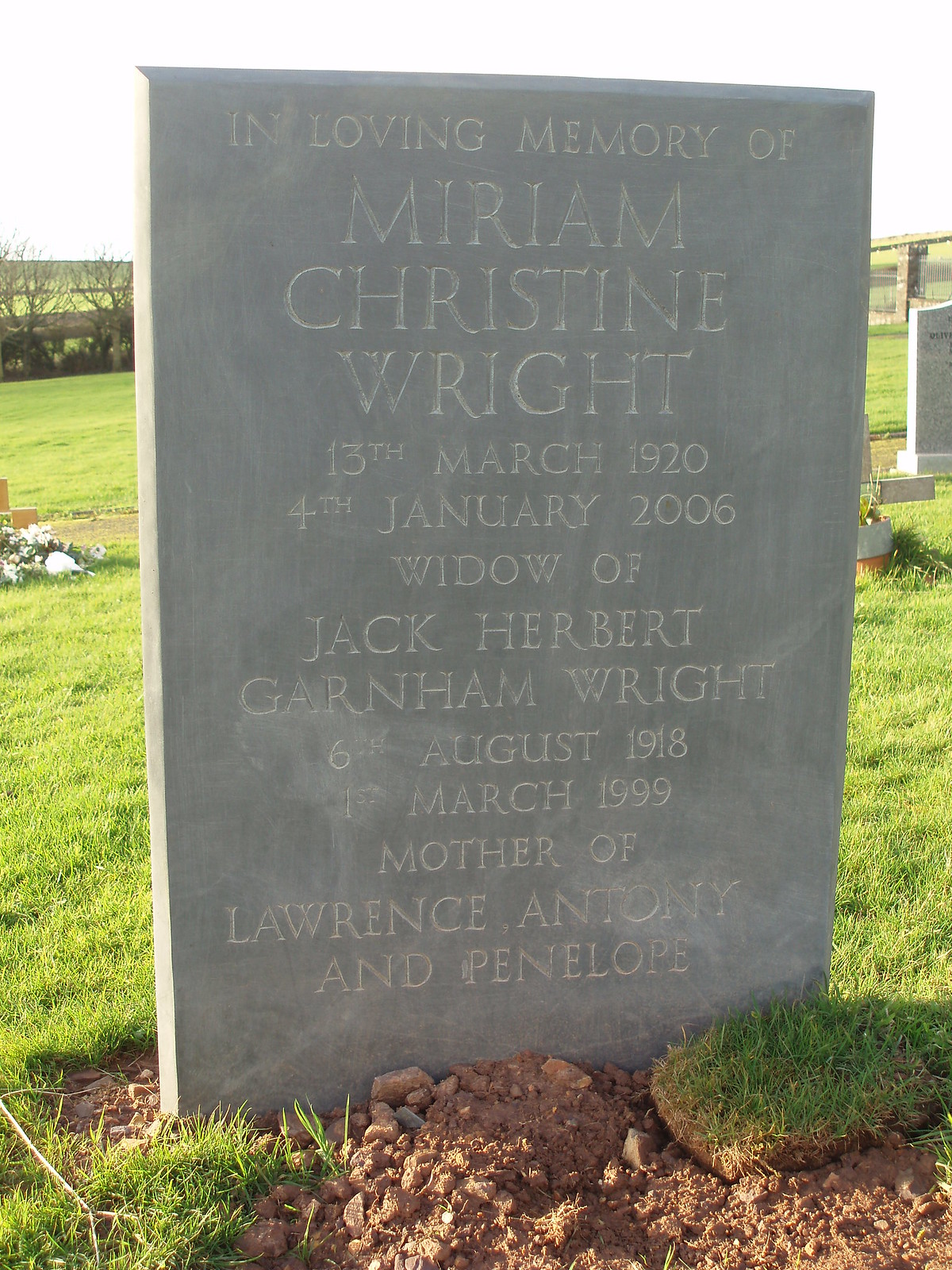In this image, a large grey tombstone stands prominently in the center of a grassy cemetery field on an overcast day, characterized by a bright sky filled with clouds. The gravestone, surrounded by patches of dirt and overturned earth indicating a recent burial, bears the inscription: "In loving memory of Miriam Christine Wright, 13 March 1920 - 4 January 2006, widow of Jack Herbert Garnham Wright, 8 August 1918 - 1 March 1999, mother of Lawrence, Anthony, and Penelope." The backdrop features sparse grass and a few other scattered gravestones, all contributing to a rather solemn and tranquil setting. The colors present are a mix of green, brown, grey, and hints of white and yellow.